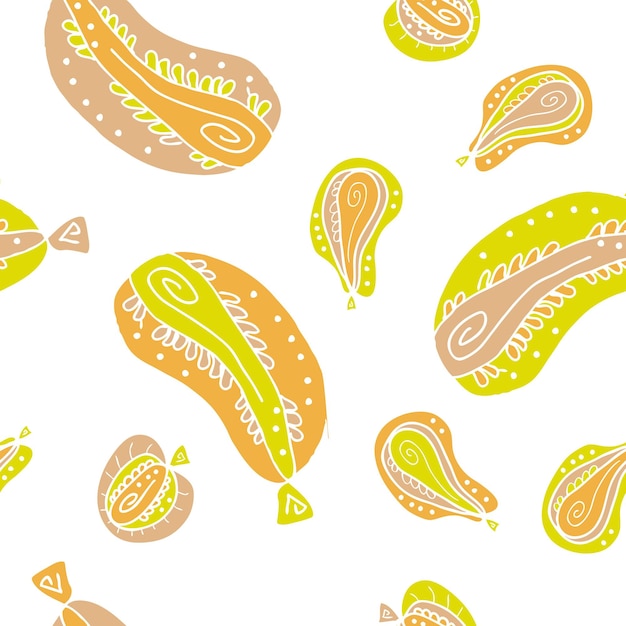The image is a lively and cheerful color illustration set against a white background, depicting various fruit-shaped forms that resemble amoeba-like creatures. These colorful shapes are primarily yellow-green, orange, beige, and brown, with some having an outer circular area and a fish-like shape within, adorned with little arm-like tentacles. The shapes are fanciful and imaginative, giving a paisley-like look with small, medium, and large sizes. Several shapes resemble pears with a greenish-yellow outer layer, a purple middle layer, and an orange teardrop center, adorned with white curlicues and polka dots. Some forms resemble apples, elongated watermelon, stingrays, or eggplants, all contributing to the vibrant, whimsical feel of this detailed and intricate illustration.